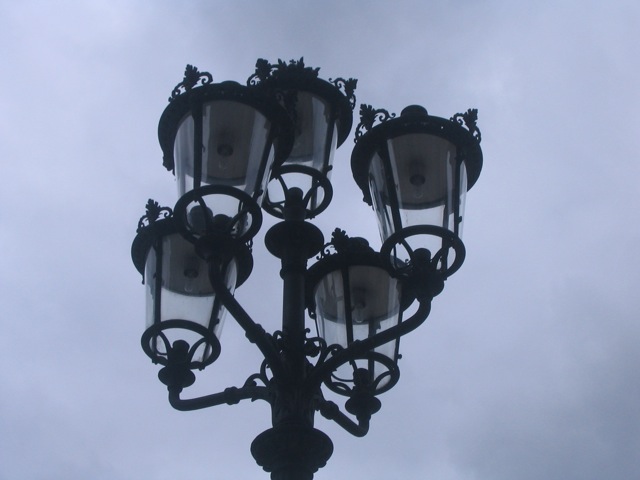This image captures an ornate lamppost viewed from below at a slight diagonal angle, set against a predominantly blue sky with patches of white clouds. The lamppost, made of what appears to be heavy-duty black metal or steel, features a central pole rising from the bottom center of the frame. From this central pole, five curved arms extend outwards and upwards at varying angles: two directed toward the back left and right, and two toward the front left and right. Each arm supports a glass lantern-like component. These lanterns are adorned with floral decorations on their lids and are held in place by black braces. Notably, the lanterns do not contain visible light bulbs and are not illuminated, despite the cloudy day. The overall aesthetic is appealing and the lamppost's detailed craftsmanship, including the decorative leaves and scrolls atop the glass sections, adds a touch of elegance to the scene.